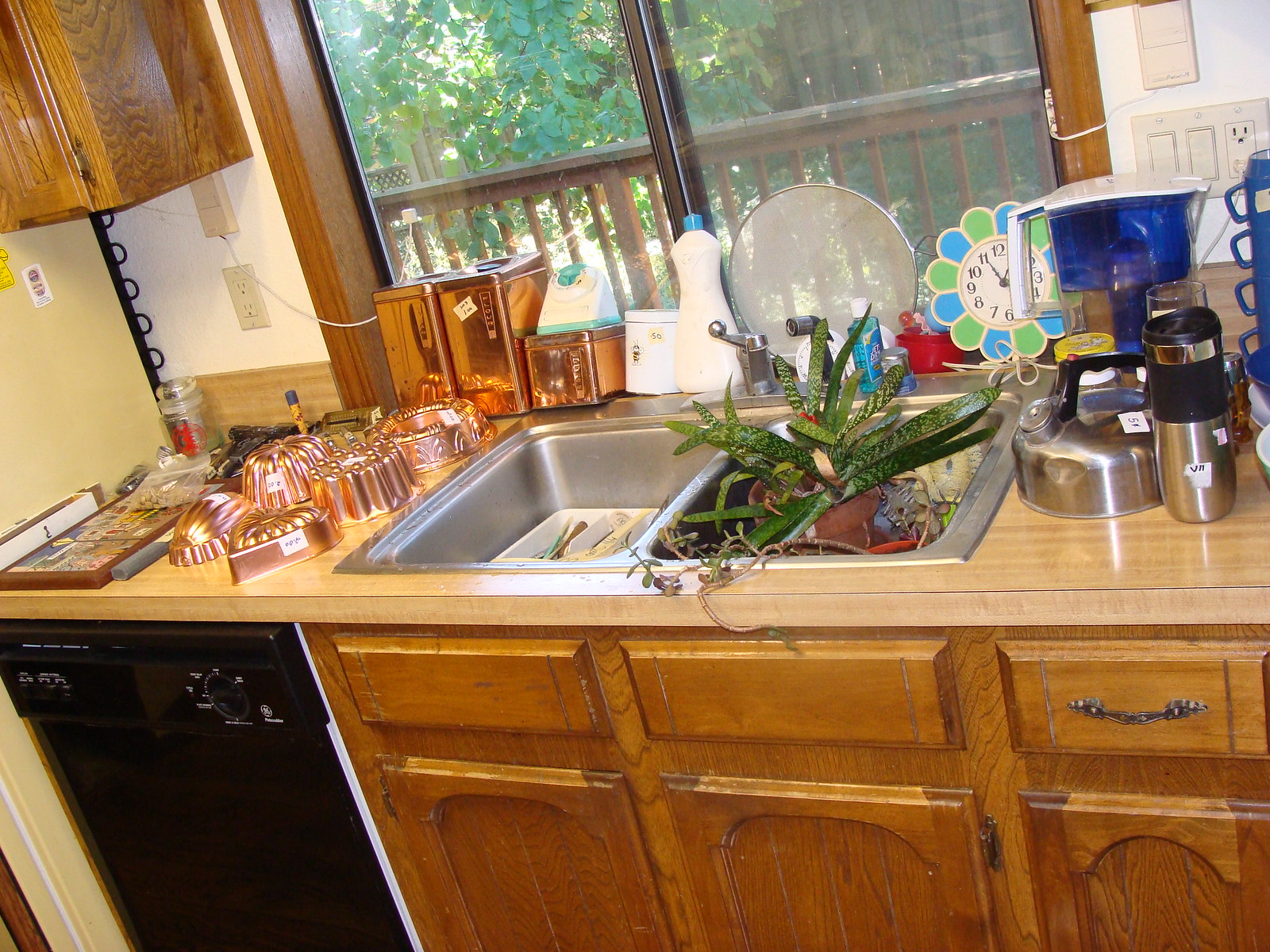In the photograph of the kitchen, there are six lower cabinets under the sink, made from old, light brown stained wood. They include three rectangular drawers, though only one drawer has a door handle. Beside these cabinets is a black dishwasher with a dial on the top right and a screen on the left side.

Above the dishwasher, five bronze-colored cake pans can be seen. Among them are heart shapes and three upside-down cake molds. Next to these, there is a white box, a picture, and a brown-gray object. A glass container and a marker with a blue cap, decorated in yellow with red zigzag stripes, are also visible. Nearby, two wooden sofa leg-like pieces are placed.

A white upper cabinet is mounted on the wall, above which is a window that opens to a view of a wooden balcony and a green tree. In front of this window, inside the kitchen, there are three tea canisters with a small white and sky-blue timer on top. Adjacent to them, there is a white canister and a white bottle with a blue cap. Leaning against the window is a pan lid used to prevent oil splashes, and next to it, a red object holding something obscure. 

A flower-shaped clock with alternating green and turquoise petals hangs nearby. A Brita water purifier stands next to a glass, a metal and black bottle, and a teal metal tea kettle. Behind these items, a glass container with a yellow lid catches the eye. 

On the white wall, an outlet with light switches is visible. From the right edge of the photo, a stack of four blue mugs on a white plate can be seen, with a green-rimmed plate slightly visible beneath. 

Inside the sink, a white tray organized with spoons, utensils, yellow paint tape, a wooden spatula, and tongs is present on the left side. On the right side of the sink, a pot containing a green succulent, along with several succulent cuttings scattered around, is evident.